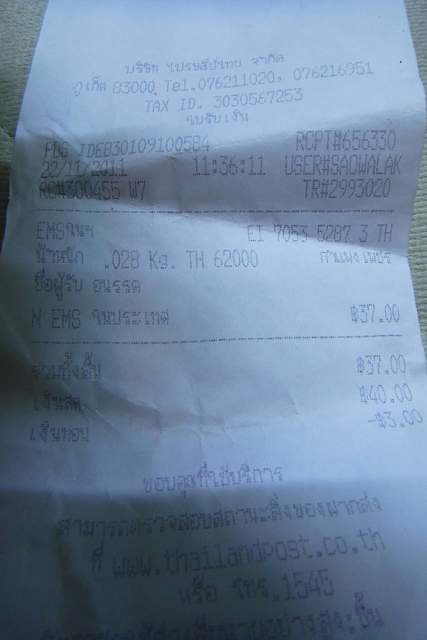The image primarily showcases a white store receipt with black text, occupying most of the rectangular frame. In the top corners, glimpses of a light-colored fabric, possibly beige, are visible, adding a subtle background element. The receipt, written in a foreign language, includes various numeric details such as the receipt number (656330), user number (SAOWALAK), and transaction number (TR 2993020). Additionally, a tax ID number, multiple prices, and the total amount are legible, although their specific values remain unspecified in the description.